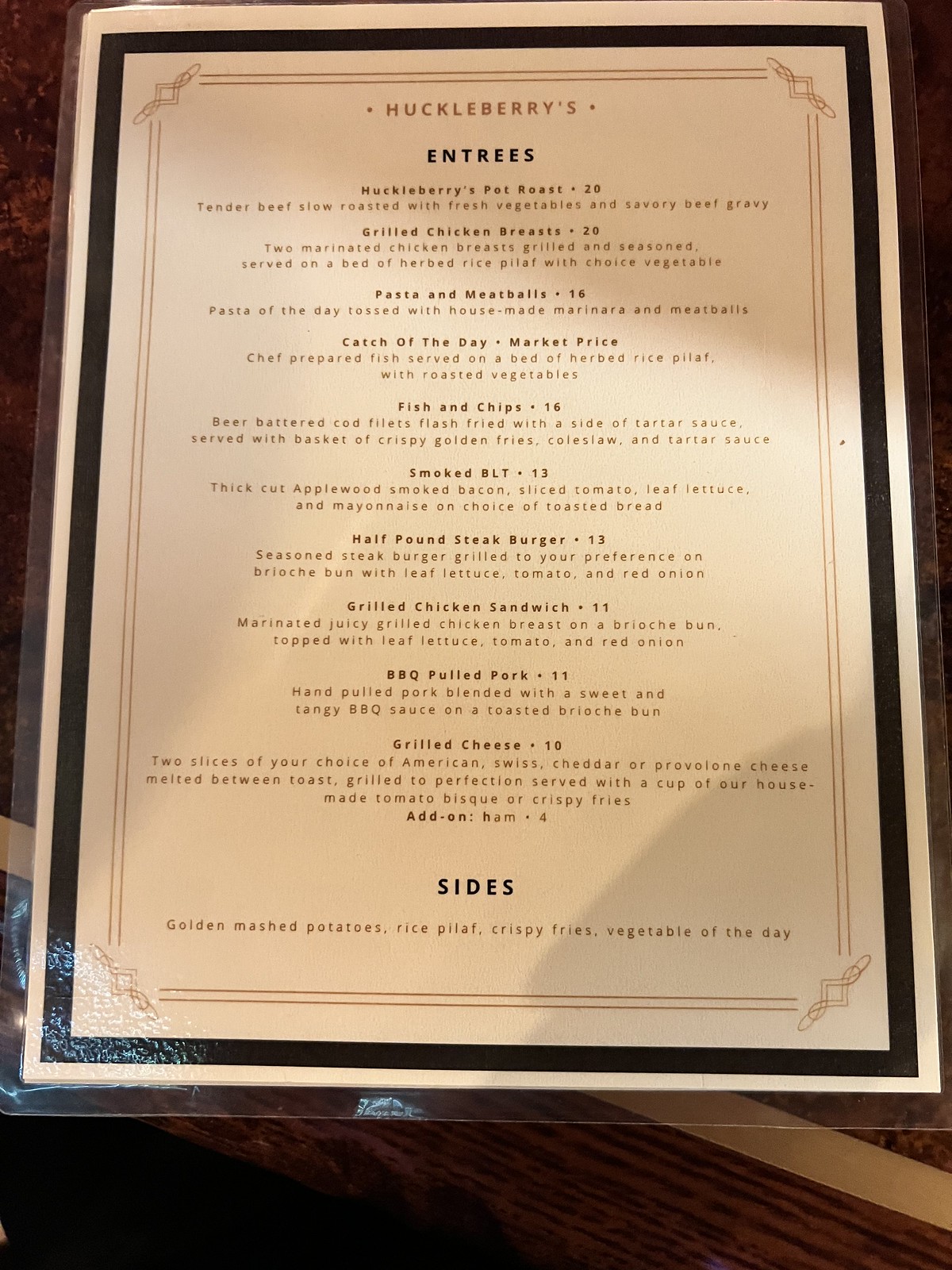This color photograph captures a menu placed on a diagonally grained wooden surface, with a distinct beige line and a small gap towards the bottom of the image. The menu itself appears to be laminated in plastic, with a clear edge at the bottom. It is illuminated by an artificial light, likely white but appearing yellowish. The menu resembles an A4 page with a narrow black rim, inside of which is a smaller beige decorative border with intricate corner elements. The name "Huckleberry's" is prominently displayed at the top in bold black text. Below this, a list of entrées is arranged in a centered format, including items like fish and chips, grilled chicken sandwich, and cheeseburger. The headings are in bold grey text, while the descriptions of the dishes are in a lighter grey, also centered. At the bottom of the menu, "Sides" is written in black text, followed by a single line describing the available sides.